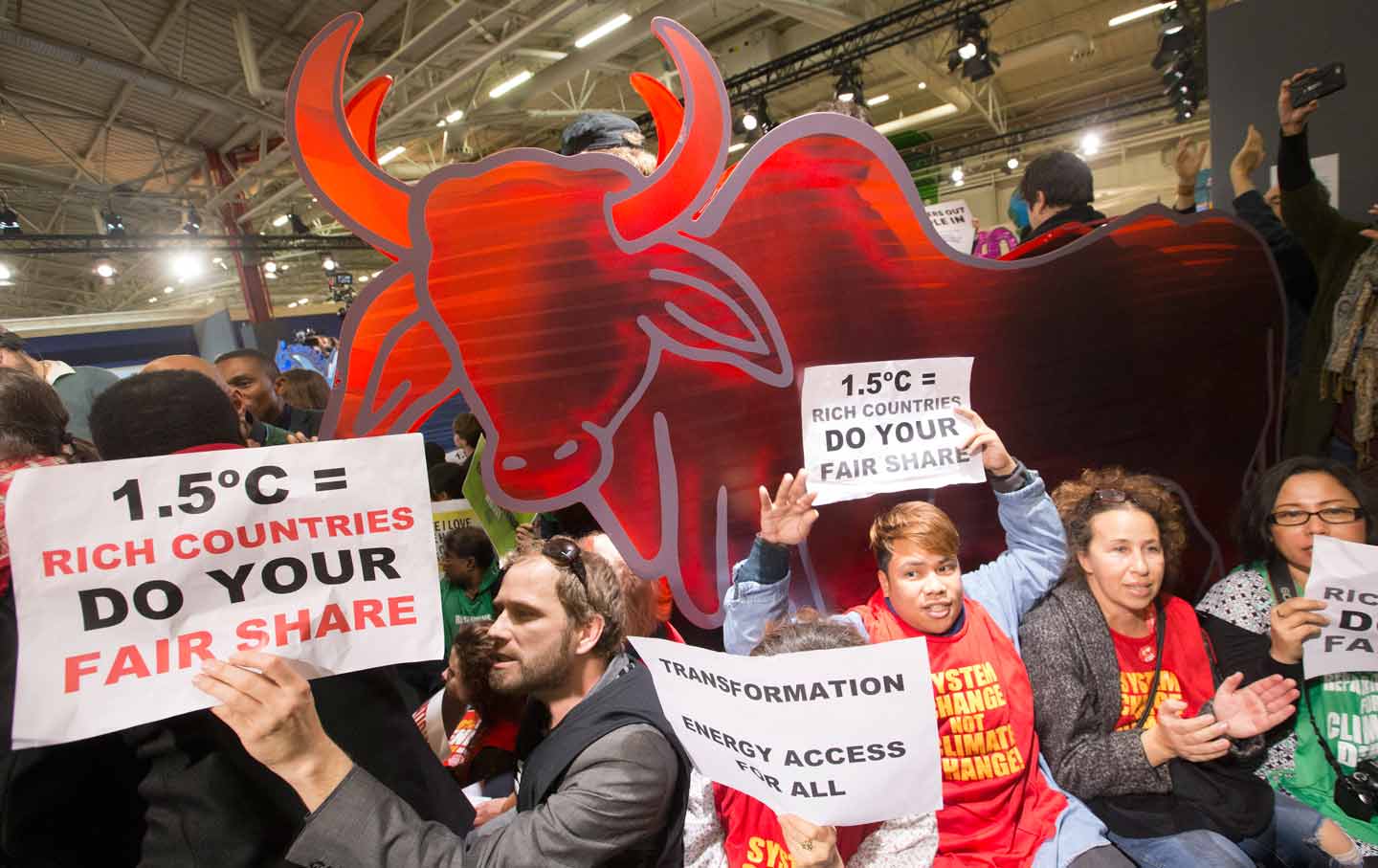This photograph, taken in an indoor setting, captures a dynamic scene of climate change protesters in what appears to be a bustling event center or conference hall. Central to the image is a diverse group of individuals, all moving from the left to the right of the frame. Prominent among them is a white man in profile, clad in a gray jacket, holding a sign that reads "1.5 degrees C equals rich countries, do your fair share." Next to him, a person donning a red apron or jumper over a white shirt holds a different sign: "Transformation energy access for all." Beside this individual stands a woman similarly dressed in a red vest bearing the slogan "System change not climate change," who is also carrying a smaller version of the 1.5 degrees C sign. Another woman in a red vest under a gray jacket is seen clapping her hands, while a woman with glasses in a green apron holds a partially visible sign displaying the letters "R-I-C-D-F-A."

The backdrop features a striking, symbolic graphic of a red bull with prominent horns moving from right to left. This powerful symbol seems to anchor the protest scene. The upper right corner of the image reveals additional participants seated in rows, possibly on benches, under a ceiling with visible lights, indicating the event's large scale. The crowded room is filled with a sea of people, many of whom are recording the event with their phones, emphasizing the significance and the energetic atmosphere of the climate change protest.